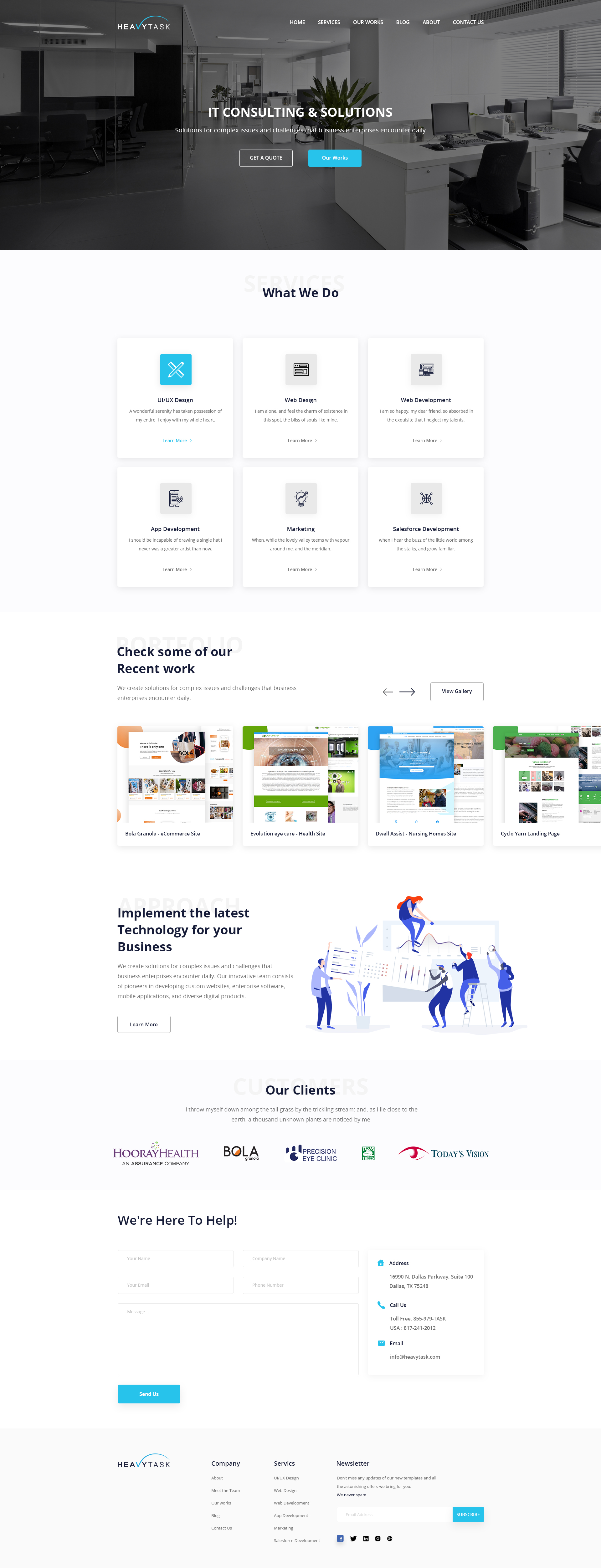The webpage presented is for a company named Heavy Task and is dedicated to IT consulting and solutions. At the top of the screen, there is a translucent black box, resembling a tinted window, that overlays an illustration of an office space displaying white desks and black chairs. Within this box, the company’s core services are highlighted: "IT Consulting and Solutions," accompanied by the tagline: "Solutions for Complex Issues and Challenges that Businesses and Enterprises Encounter."

Below this header, there are two interactive boxes labeled "Get a Quote" and "Our Works." Following these, the section titled "What We Do" features six selectable boxes, each offering a detailed description of services including Web Design, Web Development, UI/UX Design, App Development, Marketing, and Salesforce Development.

Further down the page, visitors are invited to explore some of Heavy Task's recent projects with the prompt "Check out some of our recent work." This section showcases clients like Hooray Health, BOLA, Precision Eye Clinic, and Today's Vision, indicating a focus on vision-related businesses.

Another section is labeled "Implement the Latest Technology for Your Business," with a "Learn More" button for additional details. 

In the "Our Clients" area, additional clientele is listed, reinforcing their expertise and industry reach. There is a contact form titled "We're here to help," allowing visitors to send messages or inquiries. 

On the far right, contact information is readily accessible including the company's address, phone number, and email. 

At the bottom of the page, you will find comprehensive company information, newsletter subscription options, and links to social media platforms, providing multiple channels for engagement and updates.